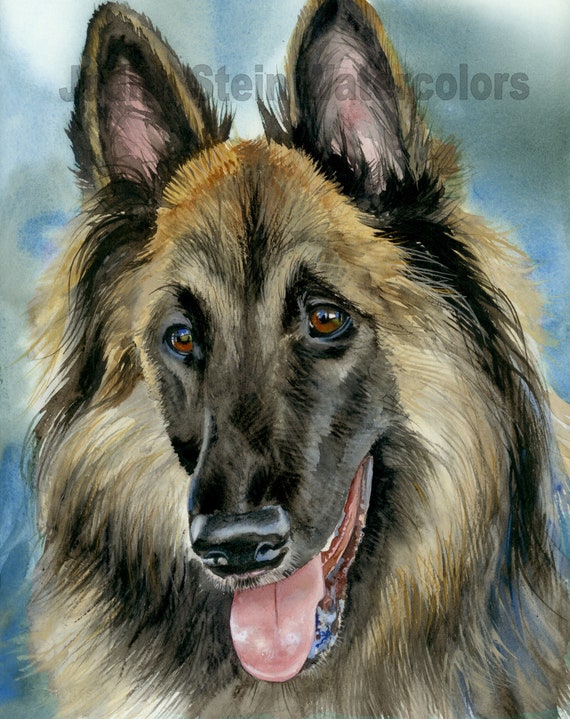This is a detailed watercolor painting by Judith Stein, depicting a friendly and playful Collie, possibly a German Shepherd mix. The dog is gazing towards the center left with an open mouth and a light pink tongue, panting cheerfully. Its ears are perked up, suggesting alertness and engagement, while its eyes are wide open and brown, with an almost reddish hue, indicating readiness for play. The dog's face features a mix of black and dark mocha brown colors, especially on the nose, and it has a Collie-like mane composed of tan, white, and black hairs. The background of the painting is light gray and blue. Notably, the image appears cropped as part of the dog's ear is cut off, and the textures are minimalistic but realistic, using mostly lines. The watermark "Judith Stein Watercolors" is prominently placed at the top, across the dog's ears.